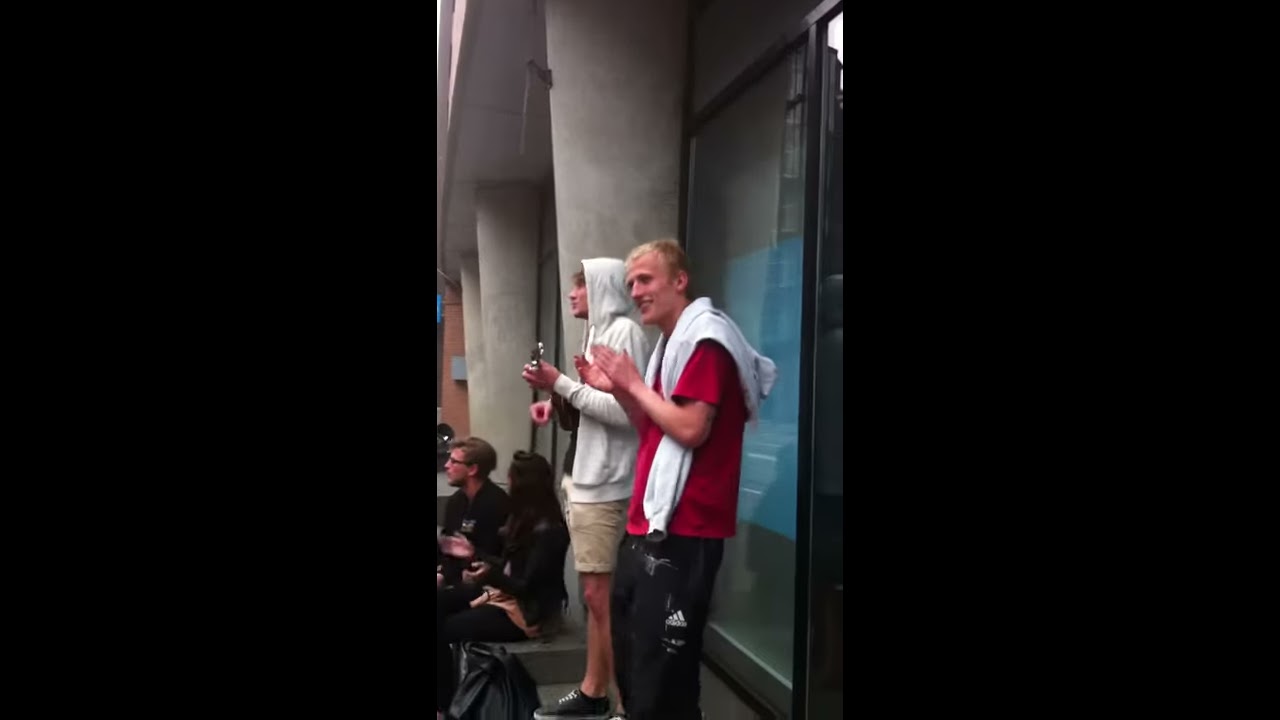In this detailed photograph, four individuals are gathered on a street side, set against the backdrop of a building that features large glass doors and gray-colored pillars. On the right, near the building's entrance, stand two young white males engaged in lively interaction. The first, with light blonde hair, wears a white hoodie and khaki shorts and is absorbed in playing a ukulele. To his left stands another young male with blonde hair clad in a red t-shirt and a white sweater draped over his shoulders. He sports black Adidas pants and appears to be smiling and clapping, adding to the upbeat atmosphere.

Further to the right, two other individuals are seated on a step. A young white male with glasses and blonde hair dressed in a black outfit sits alongside a young white female with brunette hair. The female, also dressed in black, has her head turned away and appears to be clapping her hands as well. Beside her is a black bag. Vertical black strips frame the left and right sides of the image, enhancing the focus on the group and their dynamic interaction in this outdoor setting.